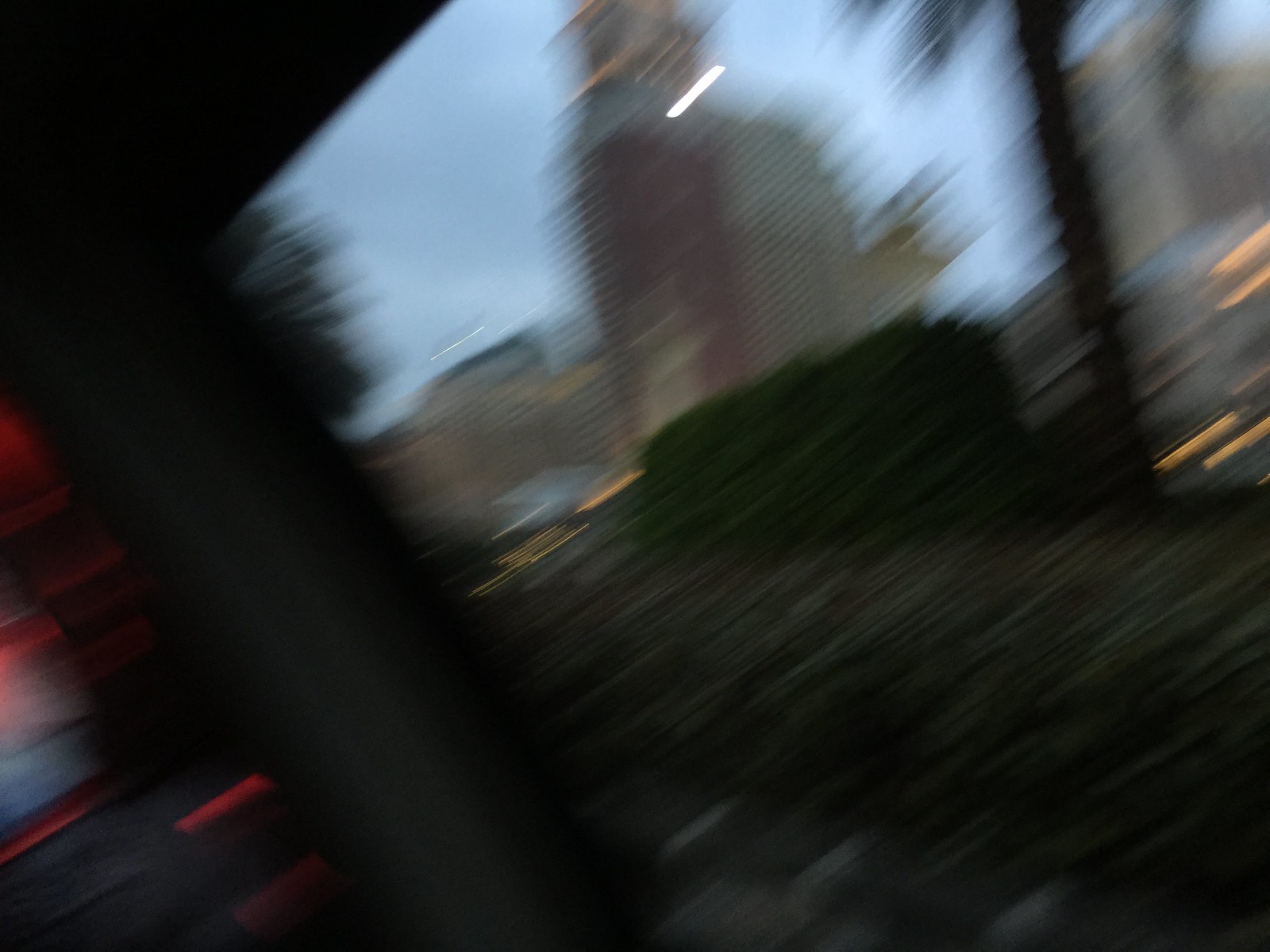This is an outdoor color photograph, likely taken at an angle while the photographer was moving, leading to a very blurry and slightly grainy appearance. The image is oriented as a horizontal rectangle and depicts a hazy scene possibly at dusk or dawn. In the background, tall, gray buildings resembling a city skyline are visible, leaning slightly to the left. The sky above is a light grayish-blue, with some clouds scattered throughout. On the top left, the photograph features a dark area that might be an overhang or ceiling. To the lower left, faint red lights streak diagonally across, appearing as short segments. The right side of the image is dominated by a dark, shadowy tree, with its black silhouette and branches reaching across the top and middle of the photo. Beneath the tree, dark green and brown hedges spread across the bottom right corner. The scene is further accented by some yellow lights and additional white light streaks near the upper right edge. There are no visible words or text in the photograph.